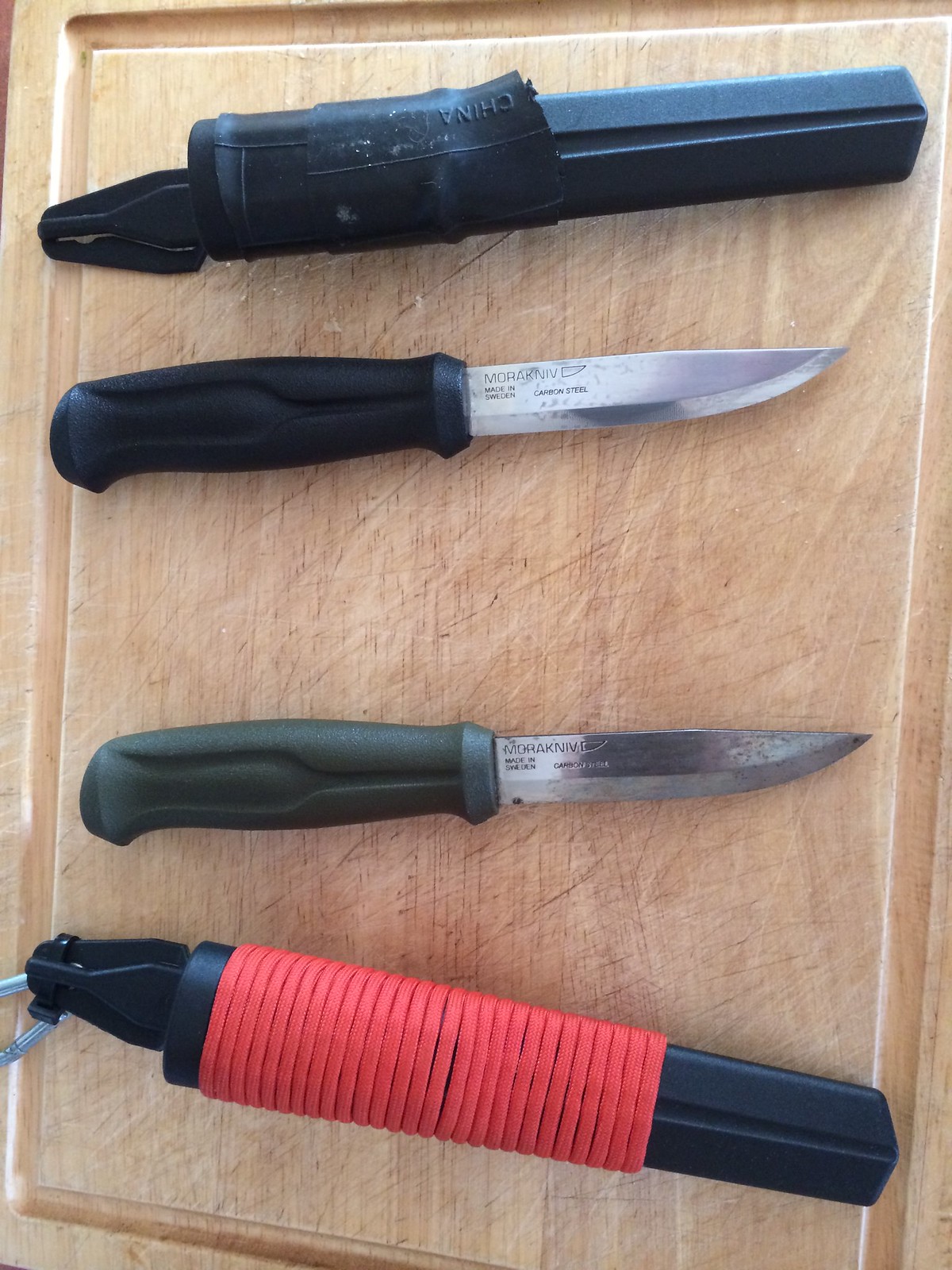This is a detailed photograph of a well-worn wooden cutting board, showing extensive scratch marks from previous use with sharp utensils. Arranged horizontally on the cutting board are four items: two knives with their respective sheaths and two butterfly knives in a closed position. The cutting board itself is a light tan color, possibly made of ash wood, with an indented groove around its perimeter.

At the top of the image is a knife sheath, made of a hard black plastic material, with "China" engraved on it and a belt mount at the top. Below this sheath is a knife with a black handle, labeled "MORAKNIV," made of carbon steel and produced in Sweden. The blade appears to be sharp and ends in a smooth, non-serrated point, although the tip shows slight rusting.

Below this knife, there is another similar "MORAKNIV" knife, also from Sweden and made out of carbon steel, but with a dark green handle. The condition of this knife mirrors the previous one, maintaining its sharpness with a pointed blade.

At the bottom of the arrangement is the sheath for the second knife, also black in color but distinctively wrapped in bright red shoelace-like cords. This sheath, too, features a belt mount at the top.

In the center of the image, there are two closed butterfly knives with black handles, positioned vertically. The hinged elements of these knives are visible, but their blades are concealed within the handles. The overall composition, viewed from a slight overhead angle, showcases both the utilitarian wear of the cutting board and the varied collection of knives placed upon it.